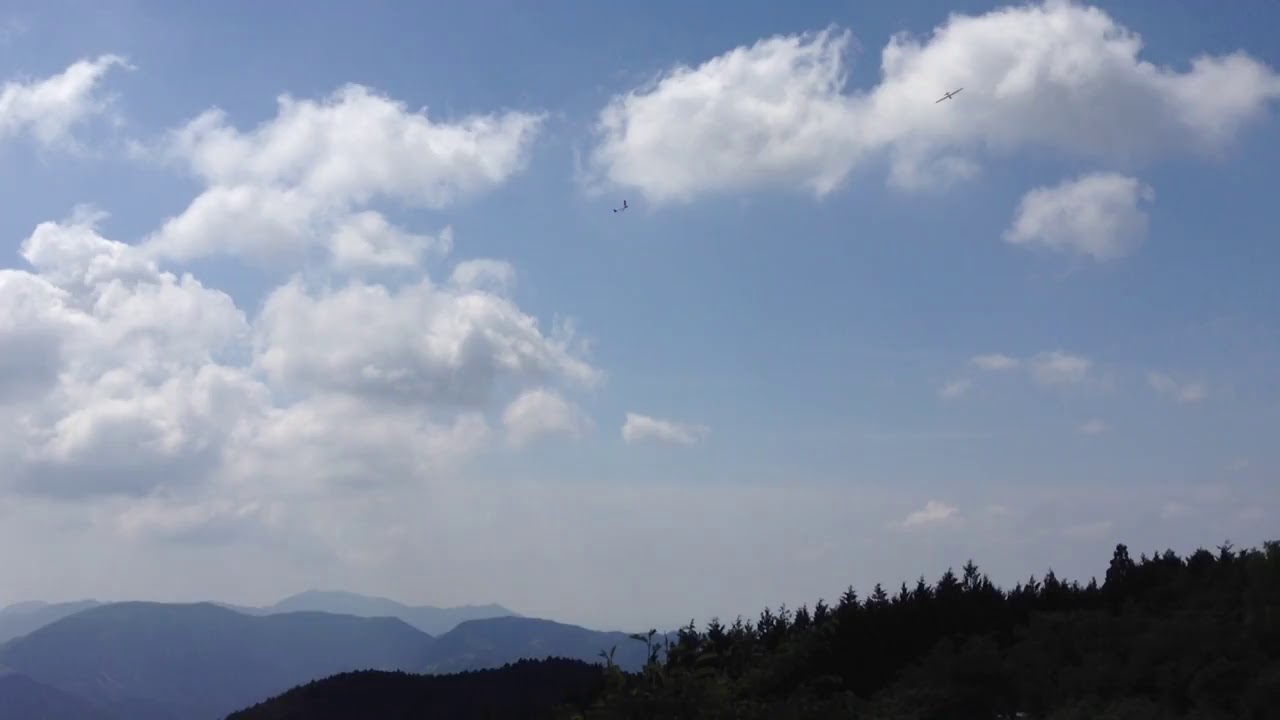This outdoor landscape photograph captures a clear, sunny day with a vibrant blue sky dotted by puffy white clouds, predominantly on the left side. The background showcases a distant, softly rounded mountain range, colored in a bluish tint, indicating their high elevation and considerable distance from the camera. In the lower right third of the image, a densely forested hill, with tall pine or evergreen trees reaching skyward, dominates the foreground. This hill's darker hue contrasts sharply with the paler, distant mountains. Notably, the image features two small, glider-like aircraft; one is positioned near the top right, angled with a wing pointing upwards, and the other is more centrally located, appearing to fly towards the first. The photograph was likely taken from another elevated hillside or a high-altitude drone, emphasizing the serene and unspoiled beauty of the natural landscape with no human presence evident.